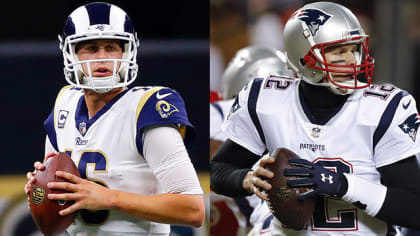This image is a horizontally aligned rectangular photograph featuring two distinct football players side by side, each occupying a square-like space. On the left side, Jared Goff is depicted in a white jersey with blue letters and sleeves, marked with the number 16 in navy with a gold outline. His Nike-emblazoned jersey and striped navy and white helmet are complemented by his bare hands, one of which secures a football as he prepares to throw. 

To the right, Tom Brady is highlighted in his Patriots uniform. His white jersey, featuring the number 12 on the shoulders, contrasts with his silver helmet adorned with the Patriots logo. Brady's left hand, equipped with an Under Armour glove, grips a football as he readies a throw, facing rightwards. Both players are captured in realistic, detail-rich portrayals, emphasizing their game-readiness and distinctive uniforms.